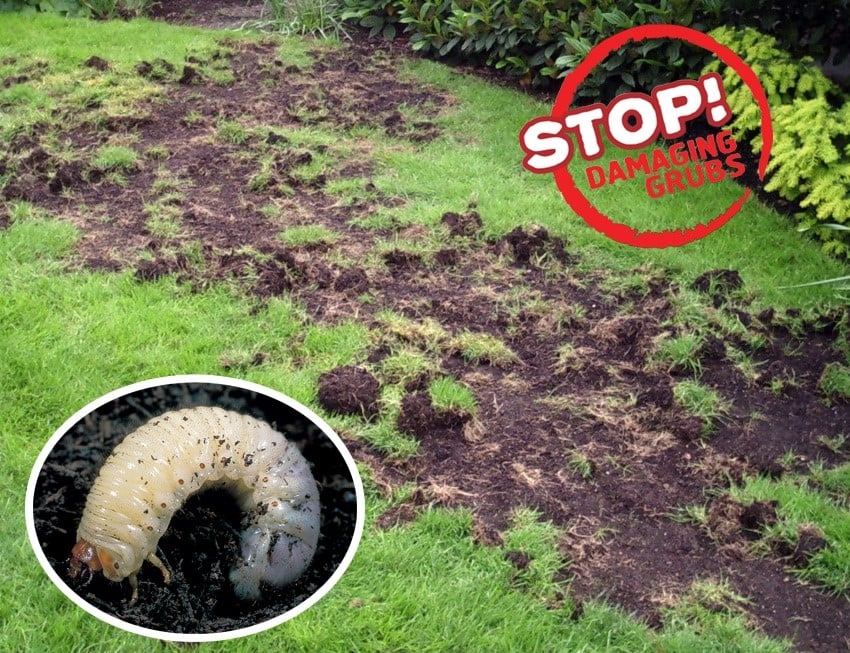The image is a public service announcement (PSA) aimed at stopping the damage to grubs. It depicts a grassy lawn severely torn up, with mud and ripped clumps of grass scattered across the surface. The scene seems to imply damage caused by digging or possibly severe mole activity, revealing the earth beneath. Prominently, there is red text in the upper part of the image that reads "STOP DAMAGING GRUBS!" with an exclamation point. In the lower left corner, there's a zoomed-in circle showing a white grub curled up on a dark brown or black background. The lawn is bordered by a flower garden, and behind the text in the upper right corner, there are visible bushes—one darker green on the left and a lighter green one on the right. The PSA highlights the importance of protecting grubs to maintain ecological balance, possibly to prevent disruption of the food chain.